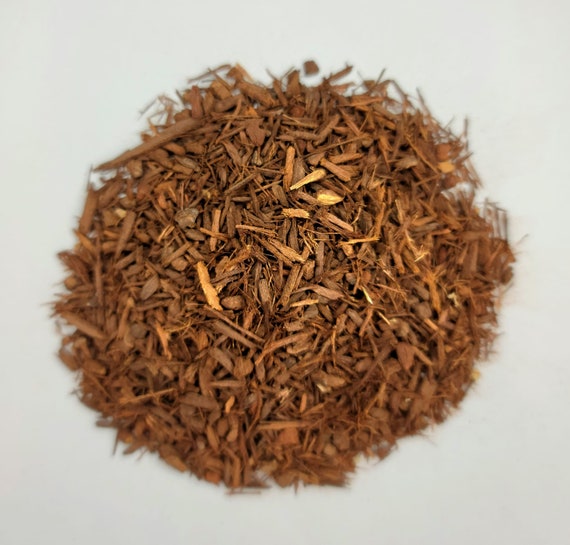The photograph captures a meticulously arranged pile of brownish-to-light brown dried leaves or wood chips, possibly resembling mulch used in gardening. The pile, approximately eight to ten inches in diameter, is set against a stark white background, which accentuates its earthy hues. The neat mound showcases a variety of chip shapes and sizes, including some pointy and regularly shaped ones, with a mixture of brown, auburn, light brown, and occasional yellowish tones. The central area of the pile is in sharp focus, revealing the texture and detail of the materials, while the edges gradually blur, adding a sense of depth to the image. The overall effect is a clear, detailed display of the dried organic material, highlighting the contrast between the subject and its white setting.